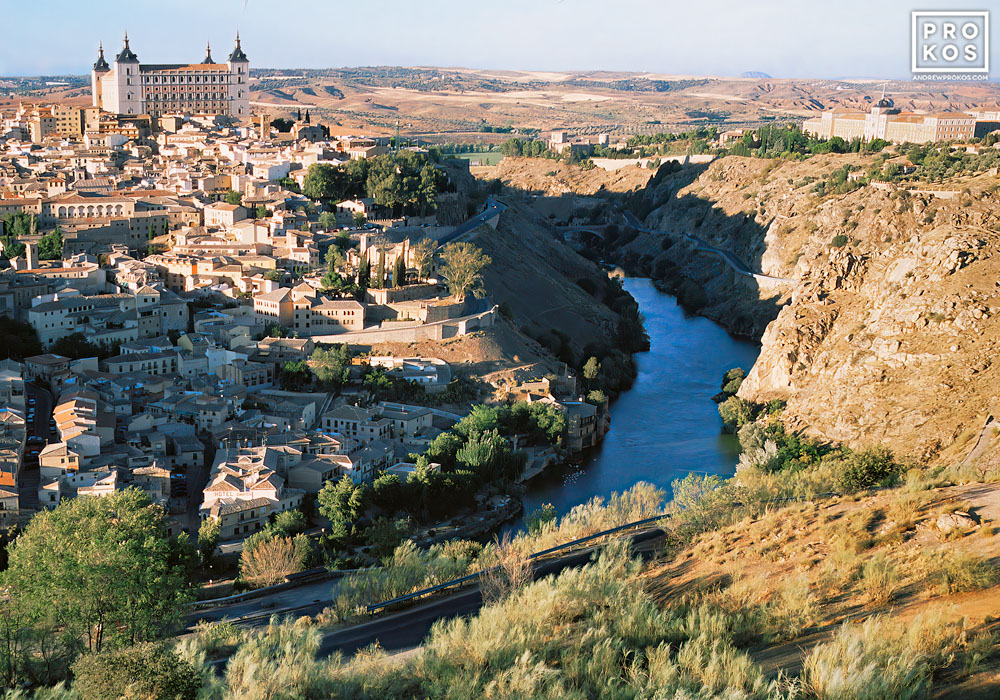This is a detailed aerial color photo capturing a picturesque town set beside a flowing river. The river winds through a gorge or ravine, flanked by rocky brown cliffs adorned with green vegetation, trees, and bushes to the right. On the left, the tops of numerous houses and buildings are visible, forming a built-up village-like area. Dominating the right side is a prominent large building reminiscent of a castle, with its cream-colored and orangey-brown facade punctuated by numerous windows, archways, and distinctive spires or crosses at its four corners. Further back, the townscape is peppered with more small buildings and another imposing structure that also resembles a castle, set against a backdrop of hilly terrain and a light blue sky. Roads and pathways weave into the town, suggesting connectivity. In the upper right corner of the image, the letters "P-R-O" with "K-O-S" underneath can be discerned, adding a touch of textual detail to the scene.